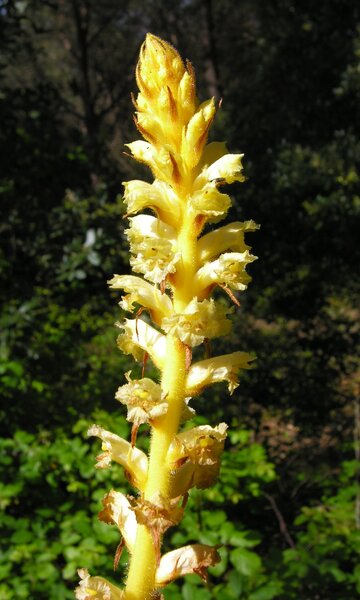This nature photograph captures a yellowish-green plant stalk dominating the foreground, extending vertically in a shape reminiscent of an asparagus stalk. The main stem shows short, stubby shoots that protrude along its length, with some shoots displaying a reddish tinge and appearing whitish due to sunlight. The top of the stalk comprises condensed flowers pointing upward. The background features a lush outdoor scene under daylight, filled with green leafy foliage, trees, and shrubs, with some hints of brown from the forest floor. The plant seems to be dying or in need of water, as evidenced by its unhealthy appearance.